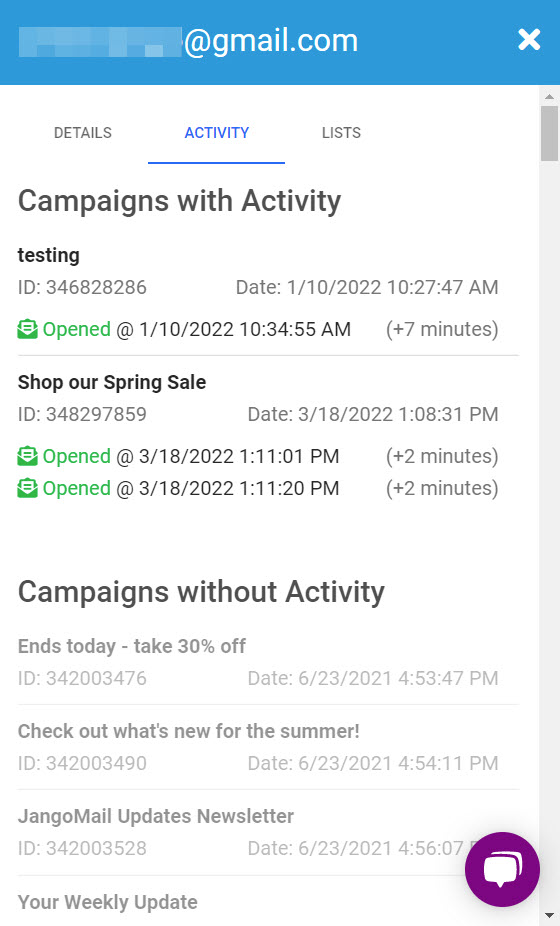This image shows the interface of an email campaign tracking tool displayed on a smartphone. At the top of the screen, there is a section obscured by a blue block with the email address ending in '@gmail.com' in white text and a white 'X' in the corner. The background of the interface is primarily white.

At the top of the display, the word "Details" is shown in gray, and next to it, the "Activity" tab is highlighted in blue with a blue underline. Further along, the "List" tab appears in gray. A gray scroll bar is visible on the right side of the screen.

Below the tabs, the interface shows a list of campaign activities with black text on the white background. Each entry in the list includes details such as the campaign's activity, testing ID, and date. For example, one entry marked with a small green square reads "Opened at 1/10/2022, 10:34:55 AM (+7 minutes)." Another entry titled "Shop Our Spring Sale" shows the ID and date, indicating it was opened and checked again two minutes later.

Entries under "Campaigns Without Activity" appear in light gray print and provide details such as deadlines and promotional information, like "Ends today, take 30% off," along with their respective IDs and dates. Other items listed include "Check out what's new for the summer," "Django Mail Updates Newsletter," and "Your Weekly Update,” each with their corresponding IDs and dates.

Towards the bottom of the screen, there is a purple circle icon beside a white quotation box layered over a smaller purple one, creating a visually distinct area within the interface.